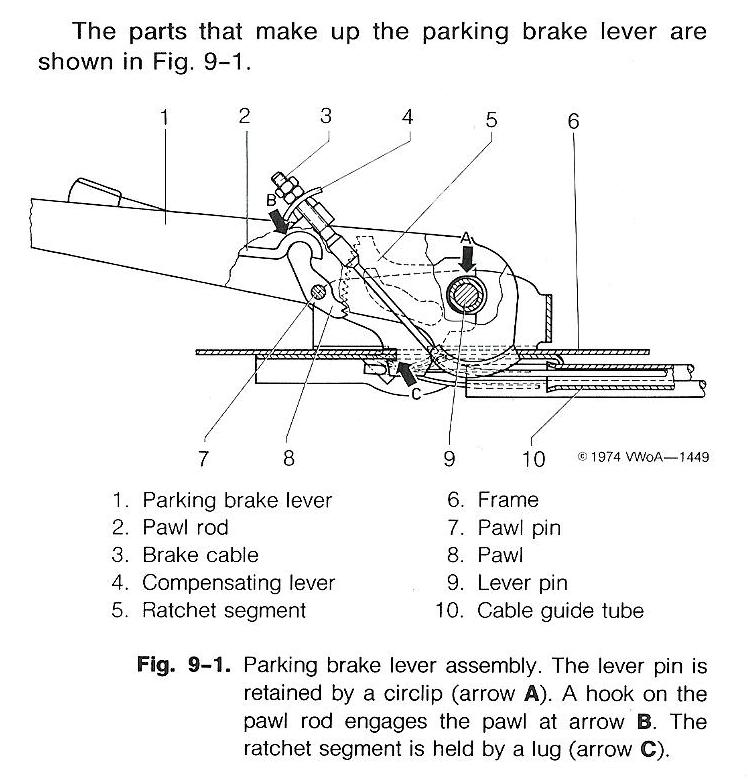The image is a detailed diagram of a parking brake lever, likely from a textbook, titled "Figure 9-1: Parking Brake Lever Assembly." The diagram is predominantly in black, white, and gray and is centered towards the top of a square layout. The accompanying text is positioned at the bottom and presented in a sans-serif font. The parking brake lever assembly is labeled with the components numbered from 1 to 10. These components include the parking brake lever, pawl rod, brake cable, compensating lever, ratchet segment, frame, pawl pin, pawl, lever pin, and cable guide tube. Key details are highlighted with bolded arrows: Arrow A indicates the lever pin retained by a circlip, Arrow B points to a hook on the pawl rod engaging the pawl, and Arrow C shows the ratchet segment held by a lug. This explanatory text enhances the reader's understanding of each part's function within the assembly. The overall style suggests an instructional or engineering-focused diagram.